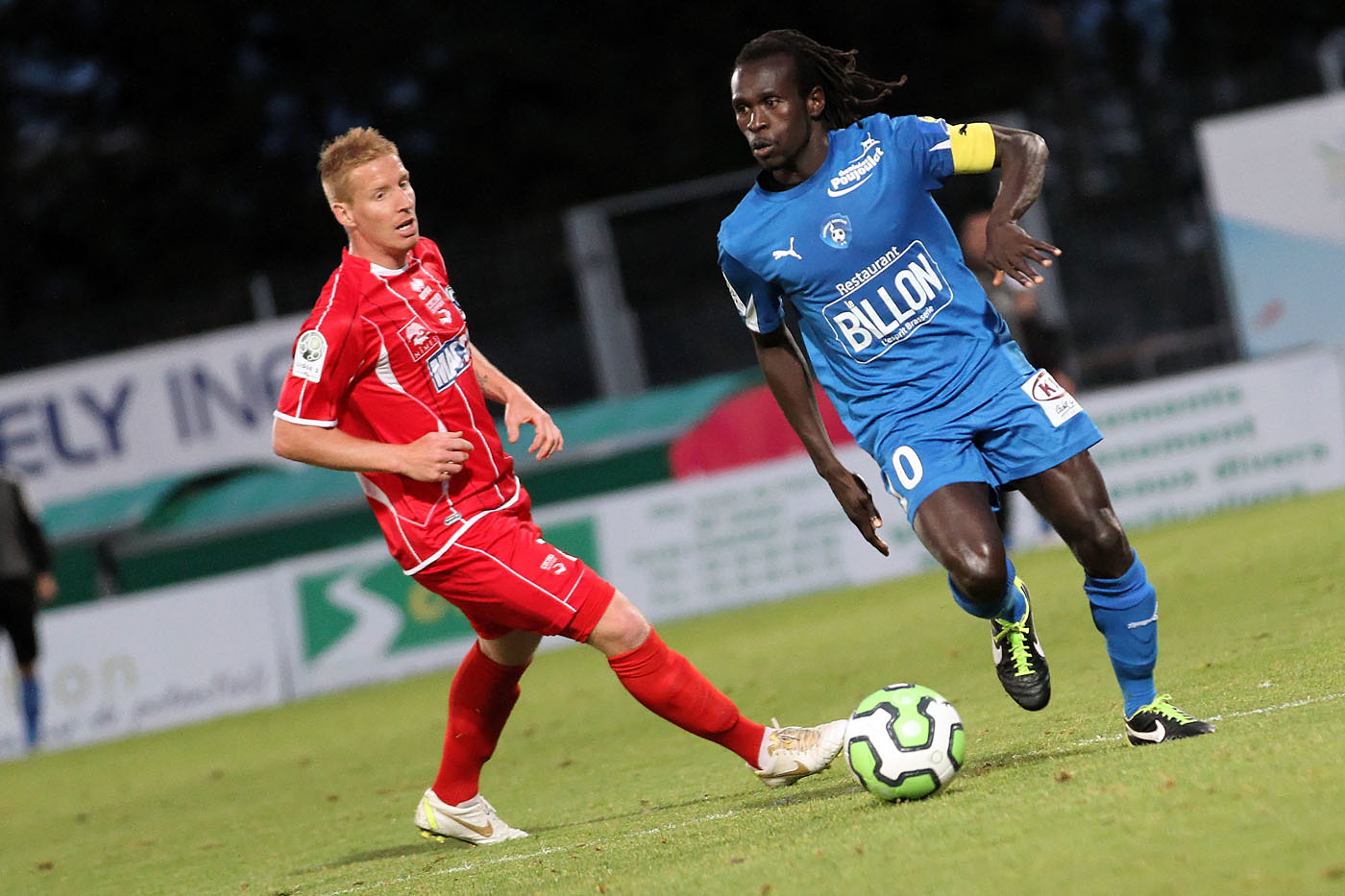In this dynamic, professional photograph, two men are captured in the midst of a soccer game on a vibrant green grass field. The focus is on an African American man in a light blue jersey and shorts, showcasing long dark hair and sporting black and green football boots with yellow laces. His jersey is emblazoned with the words "Restaurant Billion," and he wears a yellow armband. Positioned near him is a soccer ball in green, white, and black hues. Opposite him is a Caucasian man with short strawberry blond hair, donning a red and white jersey, shorts, and white boots. His mouth is slightly open, revealing his teeth as he appears to be in mid-action. In the blurred background, advertisements and possibly stands are visible, along with a partial figure suggesting a referee or another player on the sidelines. The image is slightly tilted, enhancing the sense of movement and action, depicting an exhilarating moment of the game.